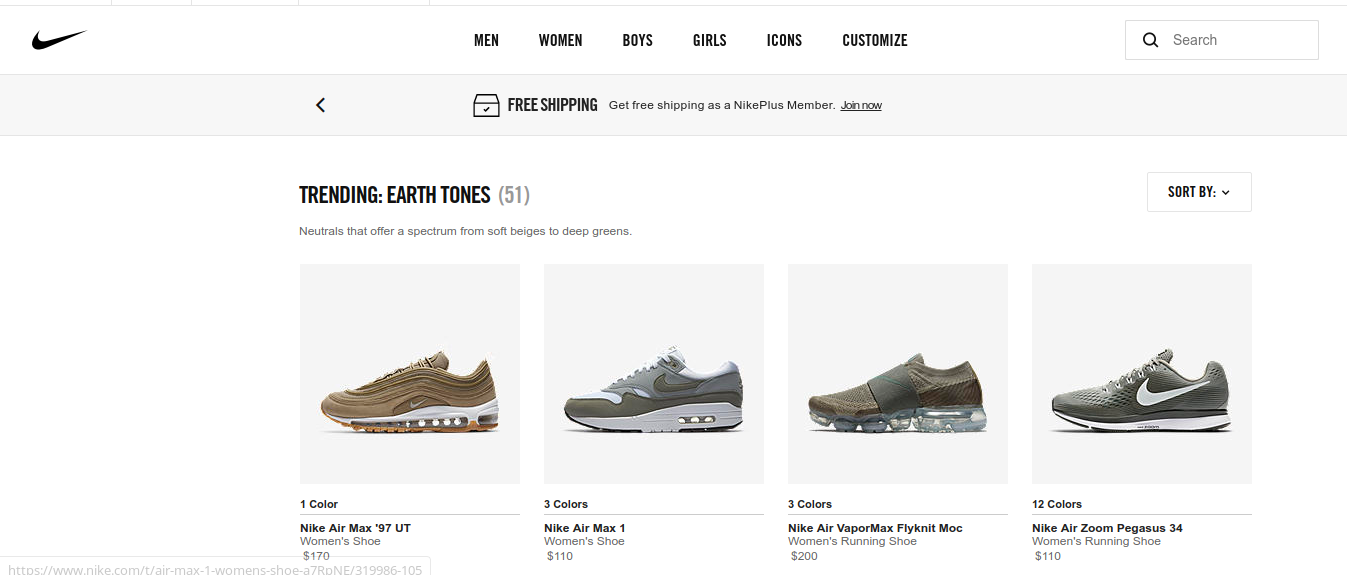A screenshot of a computer screen showcases the Nike website. The top bar of the website is white, with a black Nike swoosh logo prominently positioned in the left corner. The navigation menu offers categories such as Men, Women, Boys, Girls, Icons, and Customized, accompanied by a search icon for direct access to specific items.

Below the navigation menu, there's a gray center-justified bar featuring a back arrow on the left side. This bar contains an icon and the text "Free Shipping," with a clickable blue link to learn more about the shipping offer.

The main section of the page highlights a collection titled "Trending Earth Tones" with the tagline indicating that there are 51 items to choose from. On the right side of this section, there's an option to sort the items via a drop-down menu.

Displayed prominently are four shoe models, all available in earth tones and suitable for running or walking. The first shoe is the Nike Air Max 97 UT, available only in the color shown. The second is the Nike Air Max 1, available in three different colors. Additional shoes are also part of the showcased selection, emphasizing the earth tone trend.